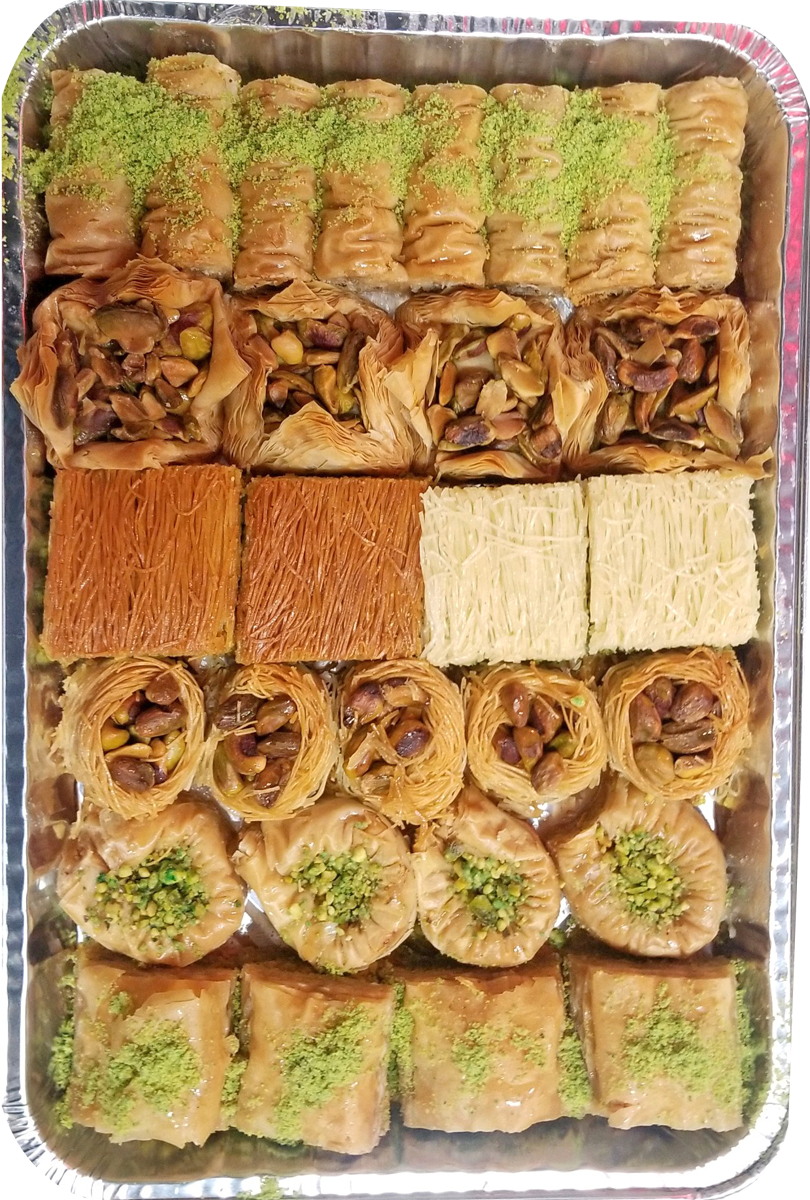A large rectangular aluminum foil serving tray, seen from a top-down view, is filled with an assortment of six types of Greek pastries. The tray, with no background or lid, appears cropped from a larger image. The pastries are arranged in six neat rows. Starting from the top, the first row features rolled pastries dusted with green pistachio crumbles. Next is a row of nest-shaped pastries filled with nuts. Following that, there is a row of traditional baklava. The fourth row showcases a different nest-like dessert with nuts in the center. The fifth row has round buns topped with pistachios, and finally, another type of baklava sprinkled with crushed pistachios occupies the bottom row. The detailed arrangement and variety suggest a carefully prepared catering platter of delectable Greek desserts.